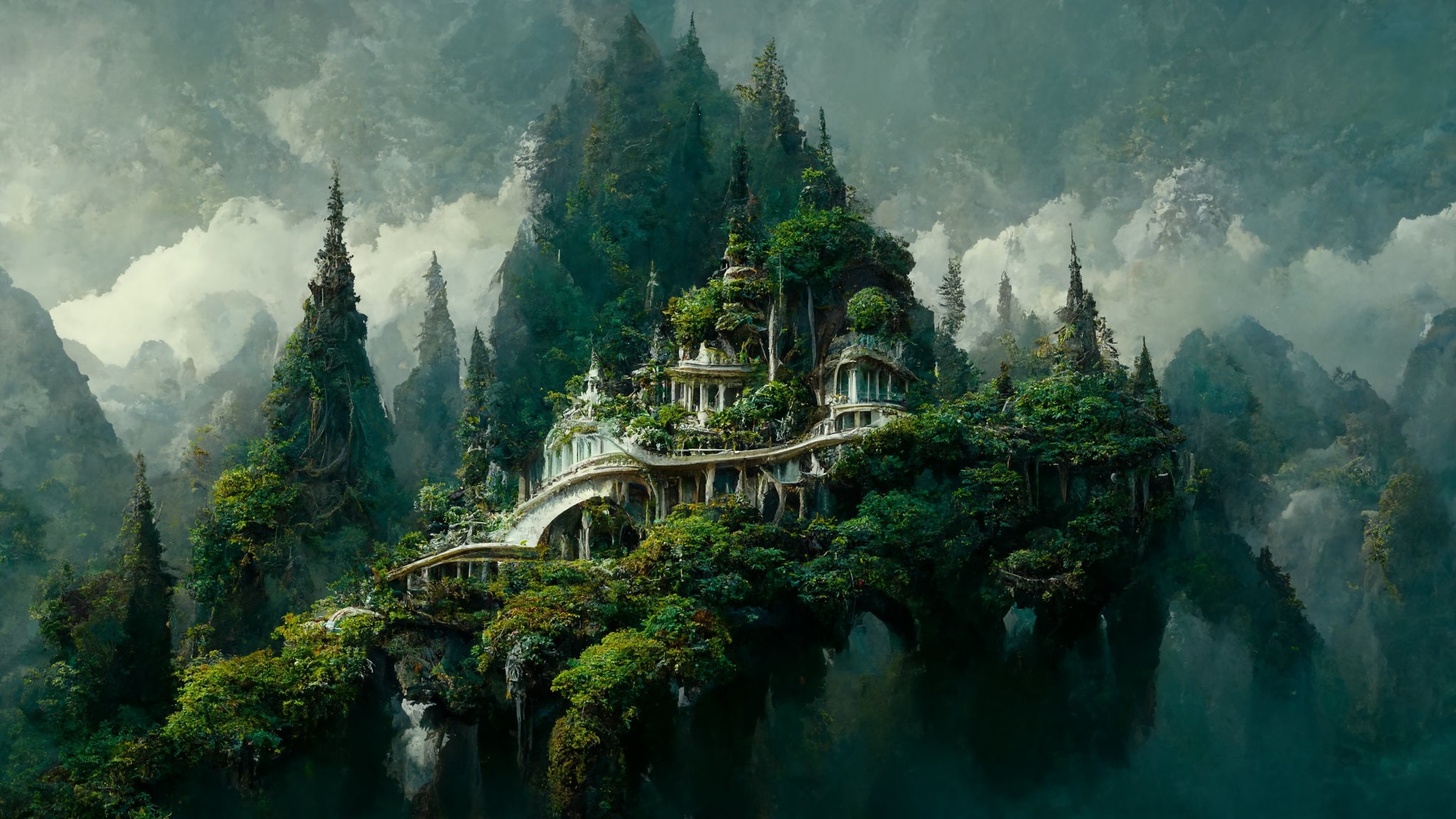The painting is a vivid and fantastical depiction of a grand, white mansion or estate nestled in a lush, mountainous landscape. The mansion, which is positioned centrally within the image, exudes an air of elegance and fantasy rather than the traditional characteristics of a castle. It is surrounded by a dense forest of tall, pointed pine trees and various other types of rich vegetation. Remarkably, trees and branches not only encircle the building but also intertwine with its structure, growing up through its levels and seemingly supporting parts of it, contributing to its mystical appearance.

The mansion is situated along a rocky cliff, and a winding trail leads up to it, with trees flanking this path. Below the mansion, a small waterfall cascades down, adding a dynamic and serene element to the scene. The background features a series of craggy mountains receding into the distance, their peaks partially obscured by a swath of fog and clouds that fill the valleys, imparting a dream-like atmosphere. Despite the heavy fog, the entire scene is depicted with great clarity and is brightly illuminated by natural lighting, further enhancing the fantastical, fairy-tale quality of the setting.